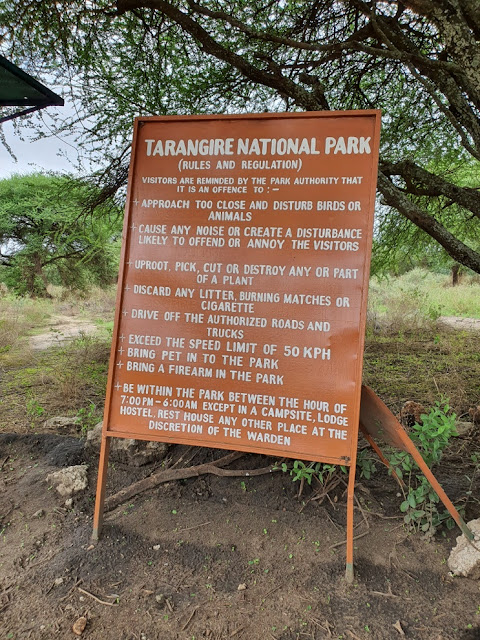The image depicts a metal sign in front of Tarangire National Park, characterized by its orange or light brown background and white text that clearly outlines the park's rules and regulations. The sign is supported by thin legs, standing about a foot above the ground in an area of bare dirt. The text emphasizes that visitors are prohibited from disturbing wildlife, creating noise, damaging plant life, littering, driving off authorized roads or exceeding the speed limit, bringing pets or firearms into the park, and staying in the park beyond designated hours except in authorized locations. Behind the sign, the setting is lush with vegetation including trees with green leaves. To the upper right of the image, tree branches with green foliage are visible, while in the far left, another leafy tree stands in the distance. There is also a hint of a roof structure in the upper left corner of the photo, adding to the scene's detailed background. The scene is captured under a clearer sky, with a fairly neutral light that suggests it may be overcast.